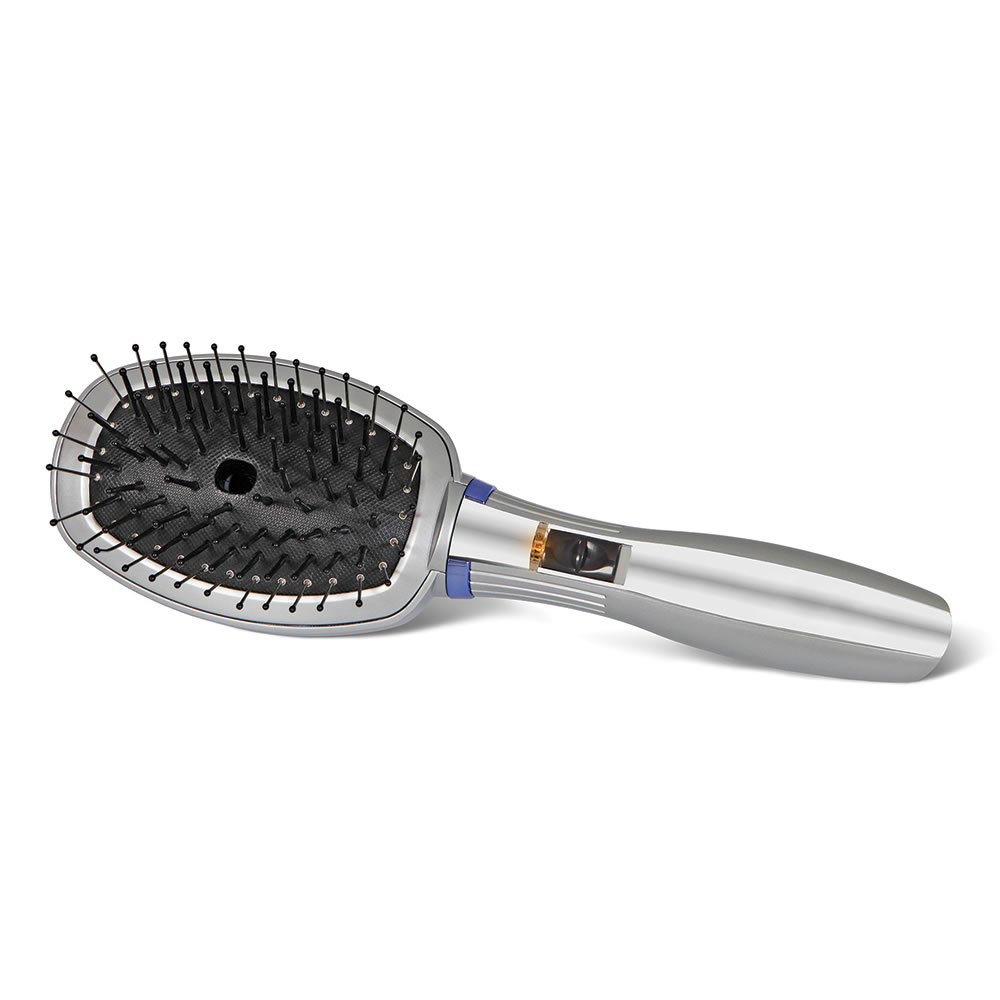This is a detailed photograph of a professional-grade hairbrush set against a white background. The brush is primarily constructed from silver metal, giving it a sturdy and solid appearance. The handle, made of the same silver steel material, features a darker gray shade on both sides and incorporates a blue rubber ring near the top, where the handle meets the brush head. This handle also includes a notable black button or switch, which is situated below an orange light, suggesting that it may be a high-tech, possibly sonic, hairbrush designed for vibration or other functions.

The head of the brush has a black soft material padding, from which the bristles emerge. Each bristle is black with a small, round black ball at the tip, designed to provide comfort during use. In the center of the brush head, there is a slightly square cutout, adding to the design's unique structure. The composition and specific details suggest this hairbrush is intended for professional use, highlighting its advanced features and durable construction.